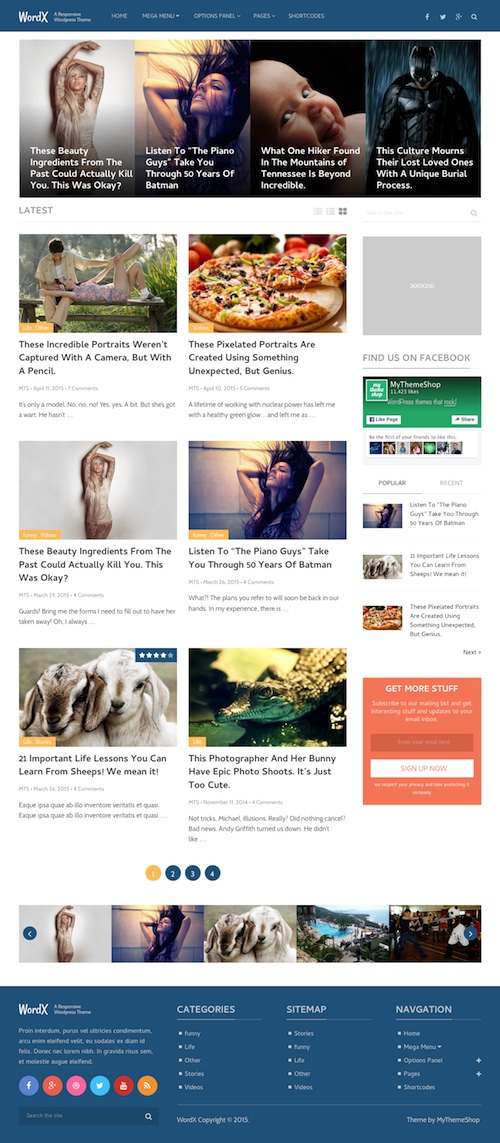### World X Website Interface

**Top Menu:**
- **Header**: "World X" prominently displayed.
- **Navigation Bar**: Home, Mega Menu, Option Panel, Pages, Shortcuts.
- **Social Media Icons**: Facebook and Twitter.

**Main Content:**
- **First Row of Images (Four Images Side by Side)**:
  1. **Image 1**: "Beauty Ingredients from the Past That Could Actually Kill You." (A compilation of antique beauty products).
  2. **Image 2**: "Listen to the Piano Guy Take You Through Many Years of Batman." (A musical journey through Batman's evolution).
  3. **Image 3**: "What One Hiker Found in the Mountains of Tennessee is Beyond Incredible." (An awe-inspiring discovery in Tennessee).
  4. **Image 4**: "This Culture Mourns Their Lost Loved Ones with a Unique Burial Process." (An exploration of a unique cultural tradition).

**Subsequent Rows (Two Columns, Three Rows):**
- **First Row**:
  1. **Left Column**: "These Incredible Portraits Weren't Captured with a Camera, But With Pencil." (Remarkable pencil drawings).
  2. **Right Column**: "These Pixelated Portraits Are Created Using Something Unexpected But Genius." (Innovative pixel art).

- **Second Row**:
  1. **Left Column**: "Beauty Ingredients from the Past That Could Actually Kill You." (Reiterated feature of antique beauty hazards).
  2. **Right Column**: "Listen to the Piano Guys Take You Through Many Years of Batman." (Reiterated musical journey through Batman's evolution).

- **Third Row**:
  1. **Left Column**: "21 Important Life Lessons You Can Learn From Sheep – We Mean It." (Life wisdom from observing sheep).
  2. **Right Column**: "This Photographer and Her Bunny Have Epic Photo Shoots – Just Too Cute!" (Charming photo shoots featuring a photographer and her pet bunny).